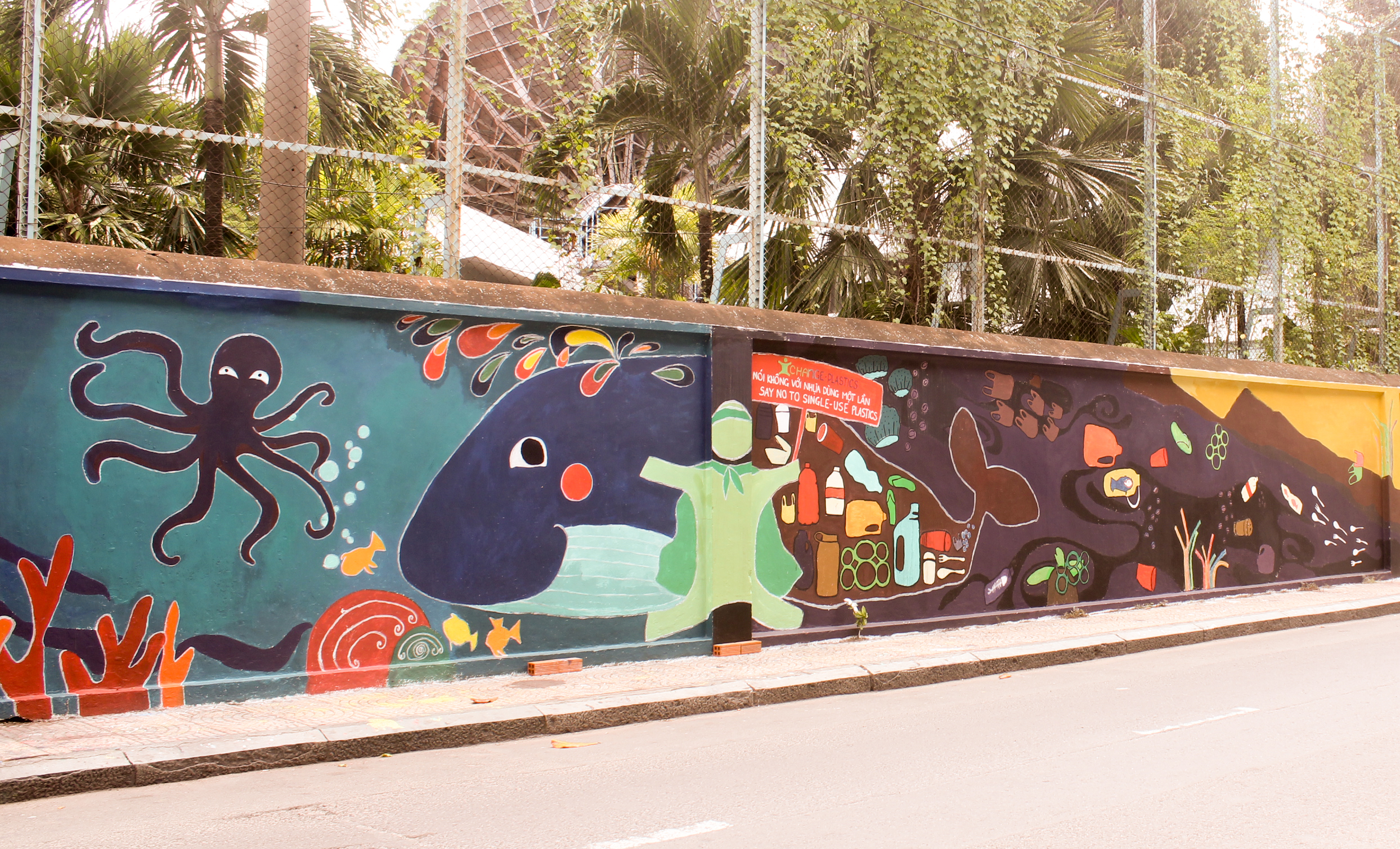The vibrant mural on this street wall presents a detailed underwater scene spanning from left to right. On the left side, the mural features a cheerful underwater environment with a black octopus, an abstract assortment of fish, the front half of a smiling blue whale, colorful coral, and playful sea lions or seals, all set against a bright blue background with bubbles rising up. At the center of the mural, there's a pale green figure donning a green cape, holding a red sign that reads "Say No to Single Use Plastic," possibly symbolizing recycling. The scene shifts on the right side to a contrasting, polluted underwater setting with a dark purple-brown hue. Here, the same whale is cross-sectioned, showing its stomach filled with plastics like six-pack rings, plastic bottles, and red solo cups. The water is murky, and the lack of coral and significantly fewer fish highlights the environmental damage. The mural sits alongside a sidewalk, with a street in the foreground and a chain-link fence and palm trees in the background.